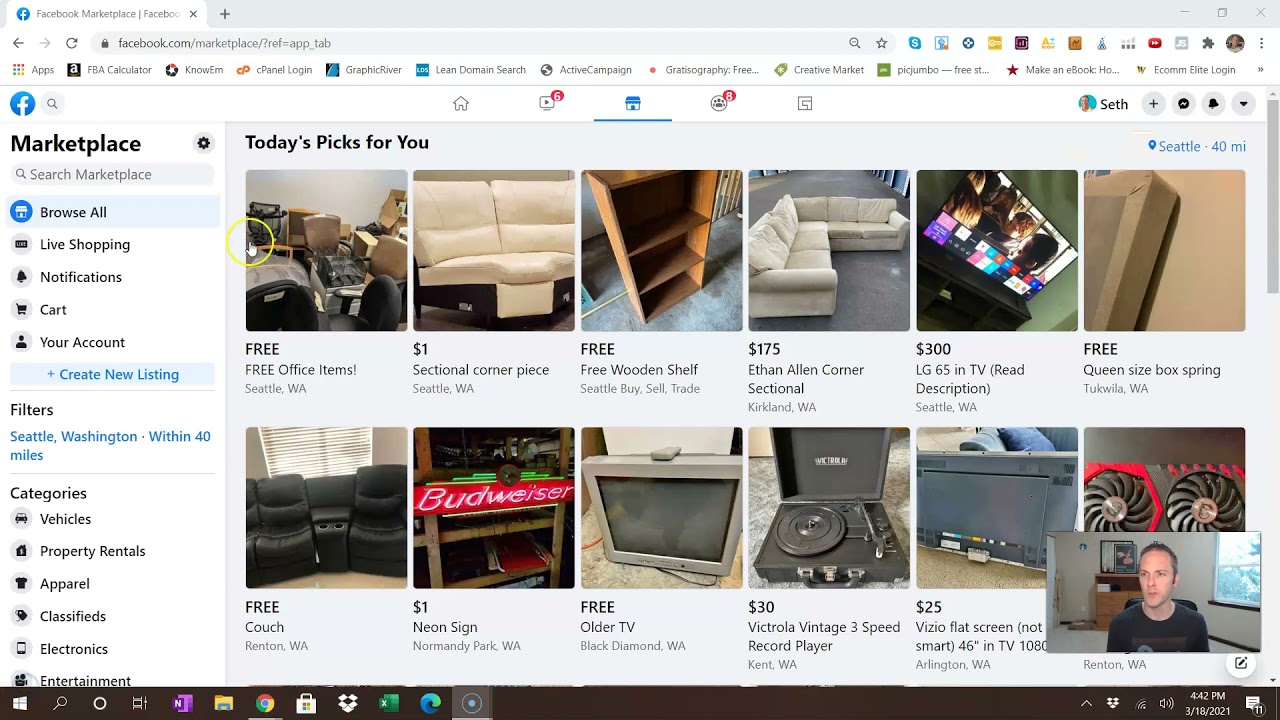This screenshot captures a complete view of a Facebook Marketplace webpage within a browser window. On the left side of the screen, the main navigation menu is visible, starting with the "Marketplace" link. Below this are various options for more specific searches, including a search bar labeled "Search Marketplace." The subsequent menu items include "Browse All," "Live Shopping," "Notifications," "Cart," "Your Account," and a prominent blue button labeled "Create New Listing."

Beneath these options, the menu continues with a "Filters" section, prominently featuring the location "Seattle, Washington," with a search radius of 40 miles, displayed in blue font. Further down, the categories listed are "Vehicles," "Property Rentals," "Apparel," "Classifieds," "Electronics," and "Entertainment."

The main content area to the right of this menu showcases "Today's Picks for You," presenting a variety of listings. These include:
- "Free Office Items," based in Seattle, Washington.
- A sectional corner piece listed for $1 in Seattle, Washington.
- A free wooden shelf in the "Seattle Buy Sell Trade" category.
- An Ethan Allen Corner Sectional priced at $175 in Kirkland, Washington.
- An LG 65-inch TV listed for $300 with a note of "re-description" in Seattle, Washington.
- A free queen-size box spring available in Tukwila, Washington.

Multiple additional listings with various items and prices are also displayed, filling out the rest of the marketplace view.